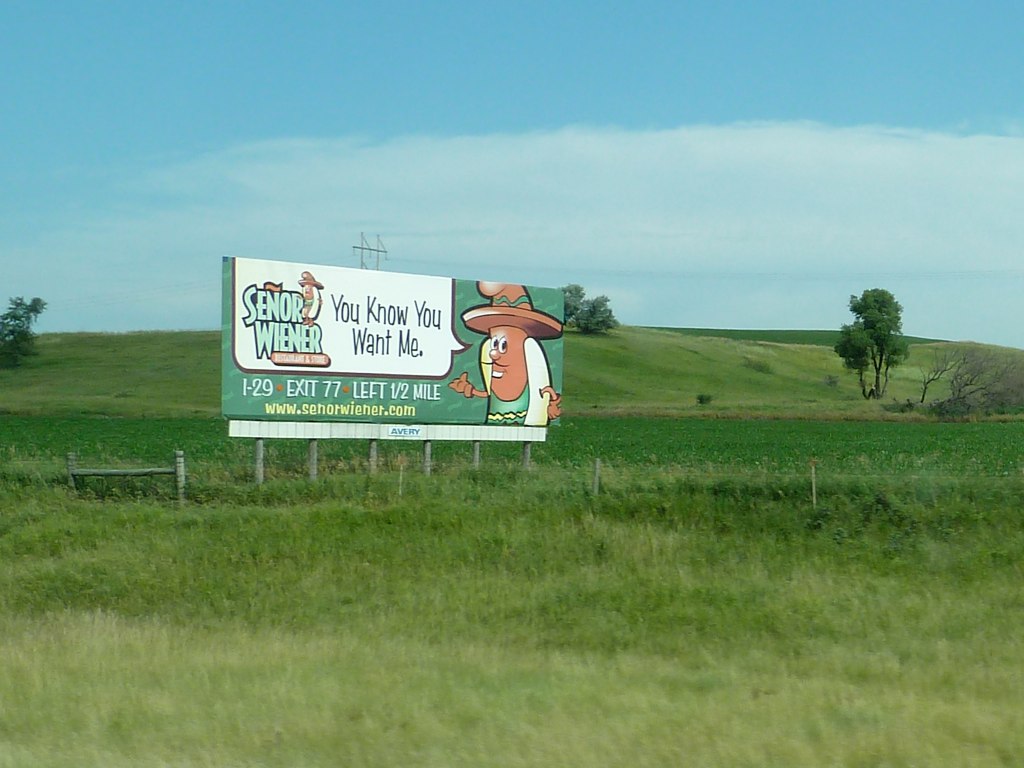In the foreground of a vast green field, there stands a large billboard sign. The grass immediately in front of the sign is a pale greenish-yellow shade, which gradually transitions to a deeper green towards the middle of the field and then fades again on the hill in the background. The hill features a variety of foliage, with a tall green tree standing prominently on the right, a tall bush in the center, and another tall bush on the left. To the right of the green tree, a few small, barren brown trees are visible. Above the hill, fluffy white clouds drift in the sky against a backdrop of clear blue. 

The billboard itself reads, "Senior Wiener, do you know me? You want me, I-29, exit 77, left half a mile, www.seniorwiener.com." The sign is adorned with a whimsical illustration of a wiener donning a sombrero hat and a mustache, exclaiming, "Hey mama!"